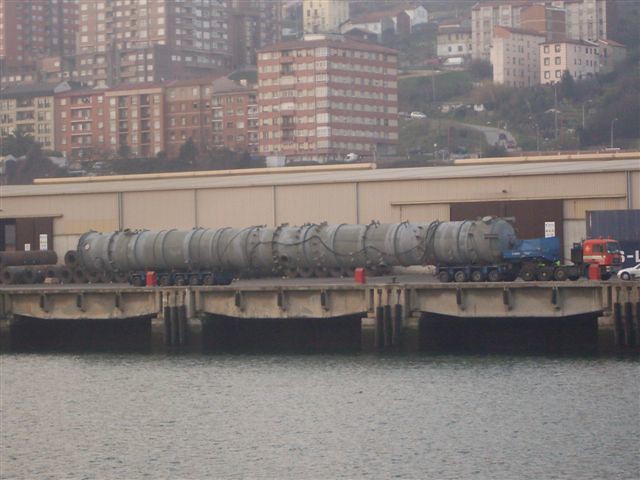In this outdoor photograph, a red semi-truck is seen hauling a massive, cylindrical, grey tank that stretches several times longer than the truck itself. The scene is set on a bridge that traverses a body of water, possibly a lake, with machinery and equipment visible in the background, suggesting some form of construction activity. The truck and its heavy load are supported by numerous sets of wheels, with seven sets at the truck’s front and another six sets at the rear of the tank. High-rise buildings of varying colors—brown, gray, white, and orange—tower in the distance, indicating a densely built urban area. The photo, likely taken during the day, seems hazy or foggy, conveying an older or low-resolution image quality, and the road appears to ascend slightly, resembling a highway on an embankment over the water.